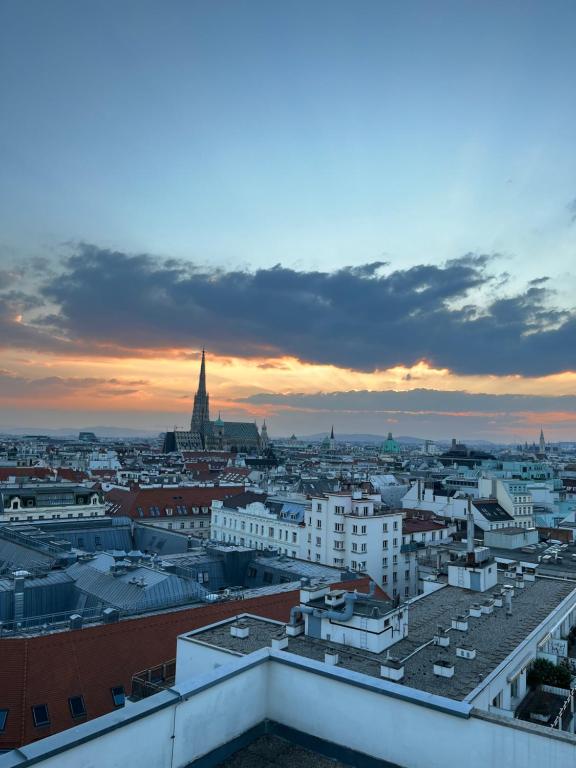The photograph, either taken at dawn or dusk, captures a bustling cityscape from a slightly elevated vantage point, possibly a rooftop. The vertically rectangular image has a sky occupying the upper third, transitioning from dark blue at the top to lighter hues as it approaches the horizon. Beneath, a large cloud, tinged with the orange and pink glow of the setting or rising sun, traverses the center of the sky from right to left. Dominating the left-center is an imposing building with a prominent, gray steeple, likely a church, with other smaller spires in the distant background.

The city below is densely packed with both white and red-brick rectangular buildings, mostly featuring flat roofs and standing no taller than five or six stories. These structures appear to be traditional European-style apartment buildings, adding to the crowded yet charming urban feel. In the far background, a green dome can be seen to the right of the main steeple, possibly another church. The horizon behind the buildings is lined with a mountain range in a blue-gray shade, lending depth to the scene. No text, people, or additional elements distract from this vivid urban tableau, encapsulating a moment of serene beauty in a bustling European city.